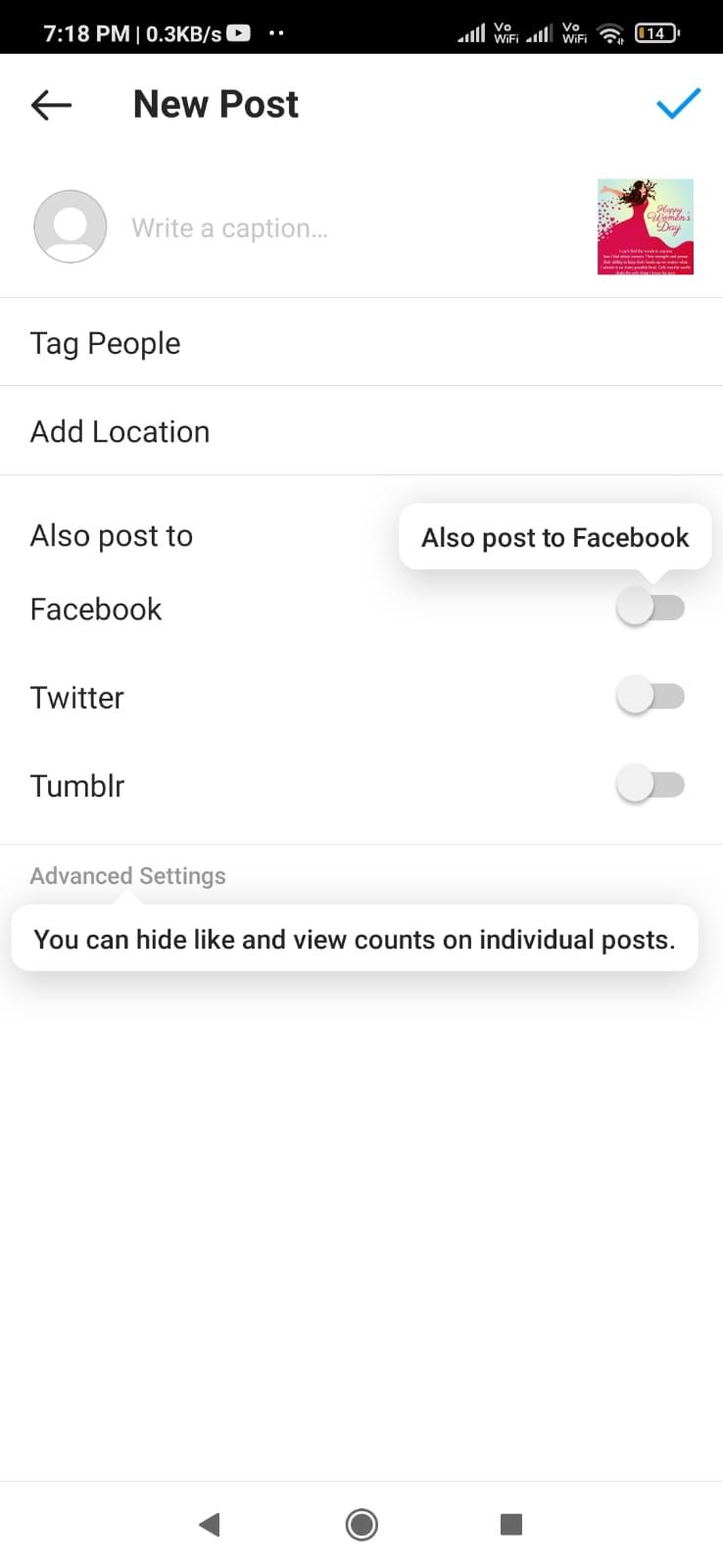Screenshot of a cellphone displaying a social media post creation screen. The status bar at the top indicates it's 7:18 PM, with data activity at 0.3 KBs, full data signal, active Wi-Fi, and a nearly depleted battery. Below the status bar is a navigation row featuring a back arrow labeled "New Post" on the left and a blue checkmark on the right. The main interface shows the text "Write a caption..." next to a thumbnail of a woman in a long red dress.

Beneath this section are options to tag people and add a location. Further down, there are toggles for additional social media platforms: Facebook, Twitter, and Tumblr, each with individual switches to share the post. Below these toggles, text indicates, "Also post to Facebook."

At the very bottom of the screen, advanced settings can be accessed, which allow the user to modify the visibility of likes and view counts on the post. The screenshot ends with a view of the phone's bottom control icons.